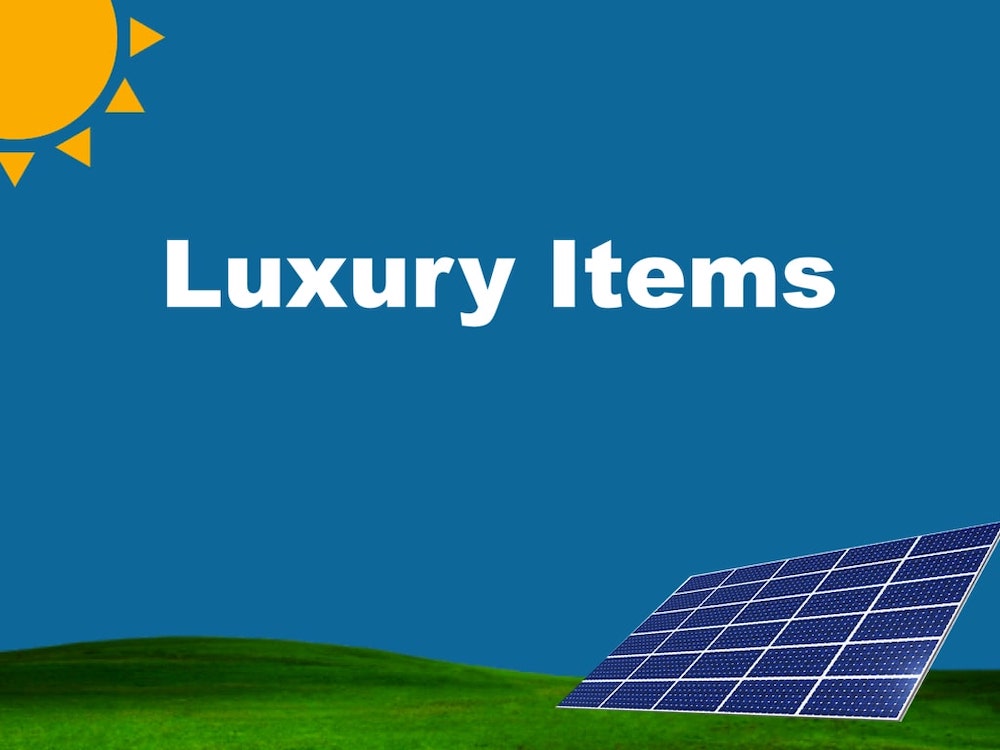The image features a blue background with several distinct elements. In the top left corner, there is an animated sun partially cut off, depicted as a quarter circle with four triangles representing its rays extending outward. The center of the image displays bold, white text stating "Luxury Items." Towards the bottom right, a grid of blue-colored solar panels is shown, angled upwards to catch the sunlight. Beneath the solar panels, there is lush, green grass, which slightly rises into a small hill on the left side. The sun, grass, and solar panels convey a harmonious blend of elements typically associated with eco-friendly and luxurious living. The overall composition suggests that this might be part of an advertisement or catalog page promoting solar panels and other environmentally beneficial items.